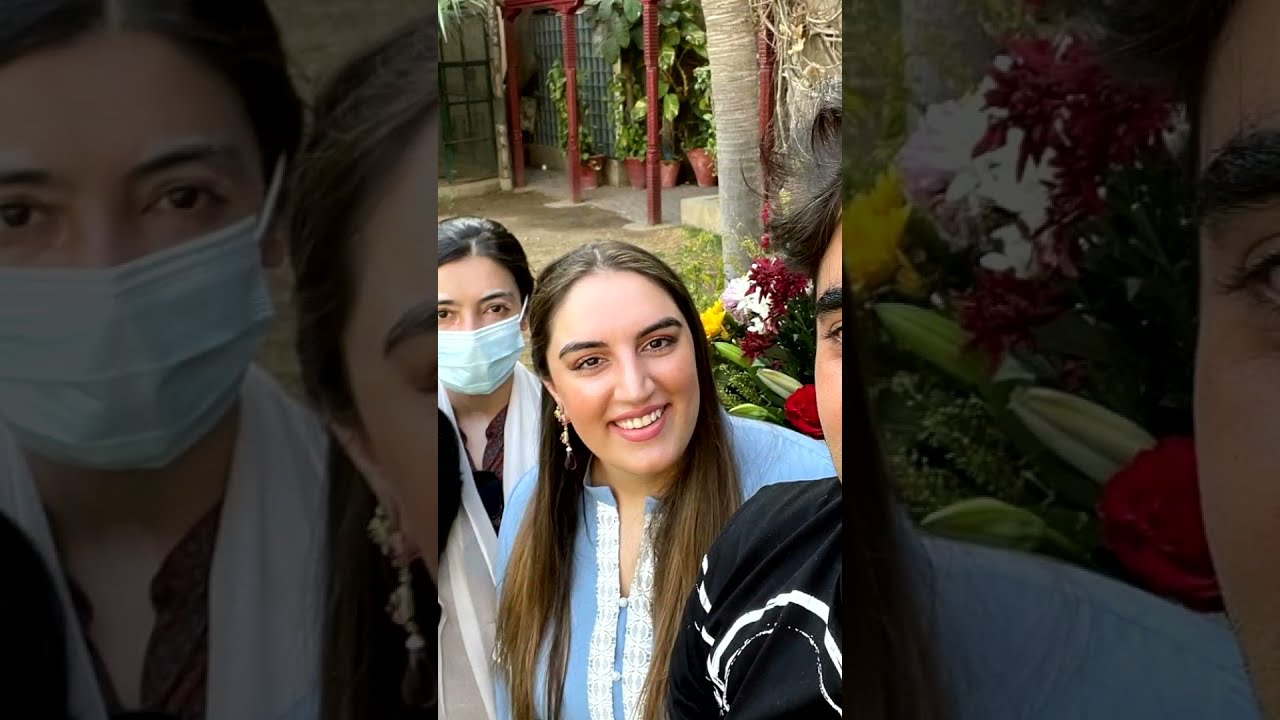In the image, positioned in a landscape format, three individuals are posing for a photograph. In the foreground on the right, there's a man partially cut off, holding a cell phone, seemingly taking a selfie. He has short, dark hair and is dressed in a black shirt with white stripes. To his left, occupying the center, is a woman in her early 20s with long brown hair. She is smiling warmly at the camera, wearing a distinctive blue top with white accents resembling an Asian style garment and an earring in her left ear. Behind her to the left, another woman stands with black hair tied back in a bun, wearing a blue surgical mask that covers her nose and mouth. She is dressed in what appears to be a cream-colored cardigan and a brown blouse or top, further accented by a white scarf. The background features a lush garden with various plants and a red fence, indicating the photo was taken outdoors.